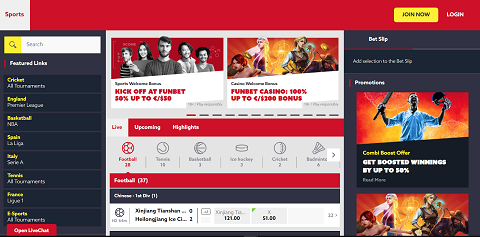The image prominently features a sports-themed promotional webpage. At the top, a large red banner encourages site engagement with the prompts "Join Now" and "Log In." On the left side, a black sidebar lists various sports categories under "Featured Links," including Cricket, England, Basketball, Spain, Italy, Trends, France, and Esports.

The central section highlights enticing offers for new users: a "Sports Welcome Bonus" offering 50% up to $50 for "Kickoff at Fun Bet," and a "Fun Bet Casino" bonus of 100% up to $100. This section is organized under sub-headings such as "Live," "Upcoming," and "Highlights," with the current featured sport being football, indicating 38 matches with 27 active players.

On the right side, there is a "Bet Slip" section with an exclusive "Symbol Boom Offer," promoting boosted winnings by up to 50%. An image of a man wearing a helmet, holding a paddle, and sporting safety goggles accompanies this section. Below this, a picture of a harem adds a visually intriguing, albeit somewhat perplexing, element to the overall layout.